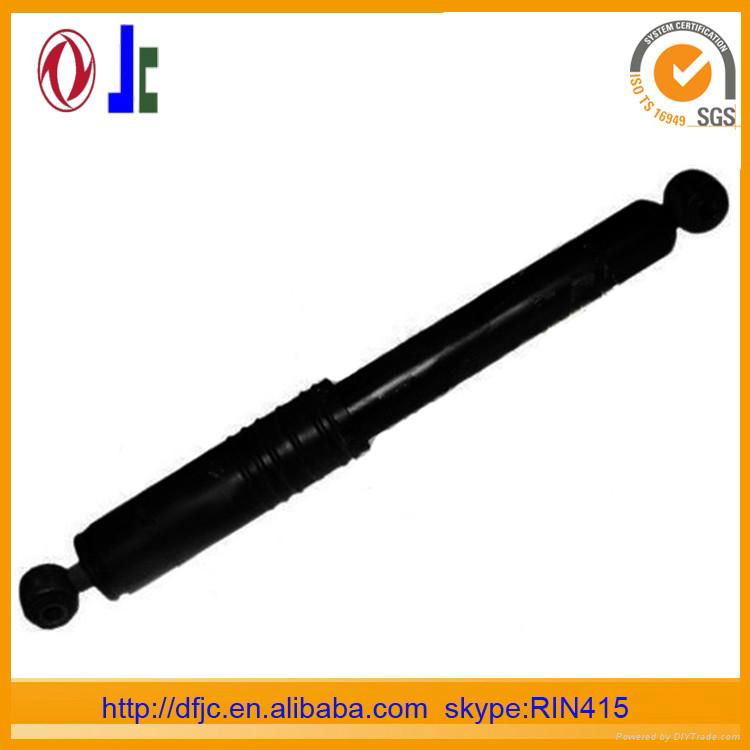This is an advertisement featuring a black rod or piston, possibly a car part, displayed within an orange-bordered layout. The top left corner showcases a logo consisting of two red blades within a red circle, accompanied by the initials "JC" in blue and green. Adjacent to this, in the top right corner, the advertisement highlights a system certification "ISO TS 16949 SGS," next to a yellow circle with a white checkmark. Beneath the product, text in blue details the Alibaba website URL "dfjc.en.alibaba.com" and a contact "Skype RIN 415," along with a note indicating the ad is powered by divtrade.com. The rod appears thin with two circles on each end, resembling a plastic baton or a hand-held item, potentially misleading as a reliable car component due to the dubious reputation of Alibaba for selling inexpensive, potentially counterfeit products.